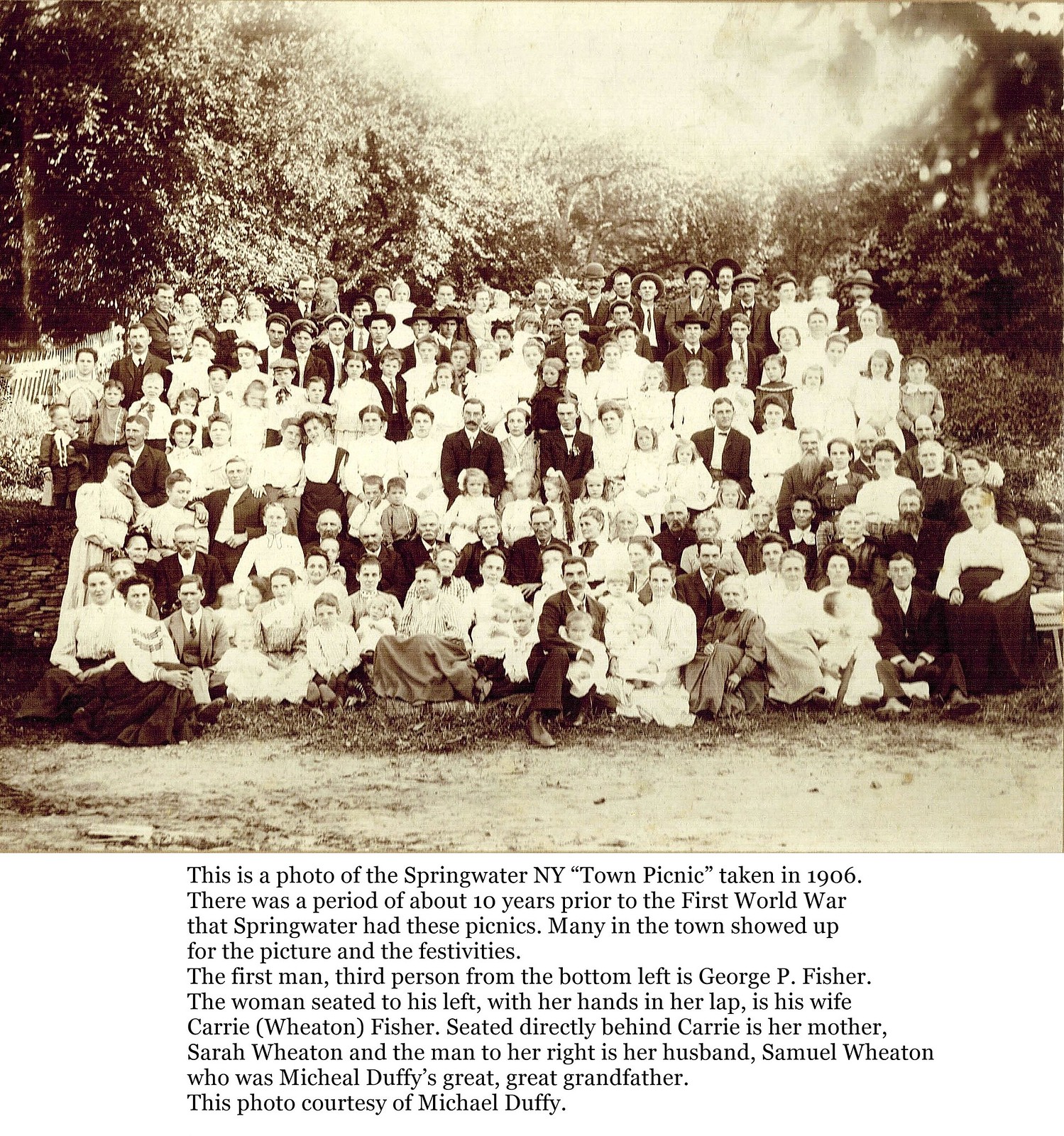The image features a vintage black and white photograph, with a noticeable sepia tint, captured in 1906. It depicts a town picnic in Springwater, New York, a tradition that took place for about ten years prior to the First World War. The photograph, which has yellowed and become grainy over time, shows light from the sky suggesting it was taken during the day, and reveals a tree line in the background. Approximately 50 to 60 men, women, and children are arranged in rows, posing in formal attire. The men are dressed in suits, many adorned with mustaches, while the women wear white or light-colored dresses, some with black skirts.

In the front row, the first man, third from the bottom left, is George P. Fisher. To his left, seated with her hands in her lap, is his wife, Carrie Wheaton Fisher. Directly behind Carrie sits her mother, Sarah Wheaton, and to the right of Sarah is her husband, Samuel Wheaton, the great-great-grandfather of Michael Duffy. The lower part of the image contains text, providing details about the photograph and noting that it was courtesy of Michael Duffy. This historical snapshot captures a cherished community event that brought the town of Springwater together over a century ago.